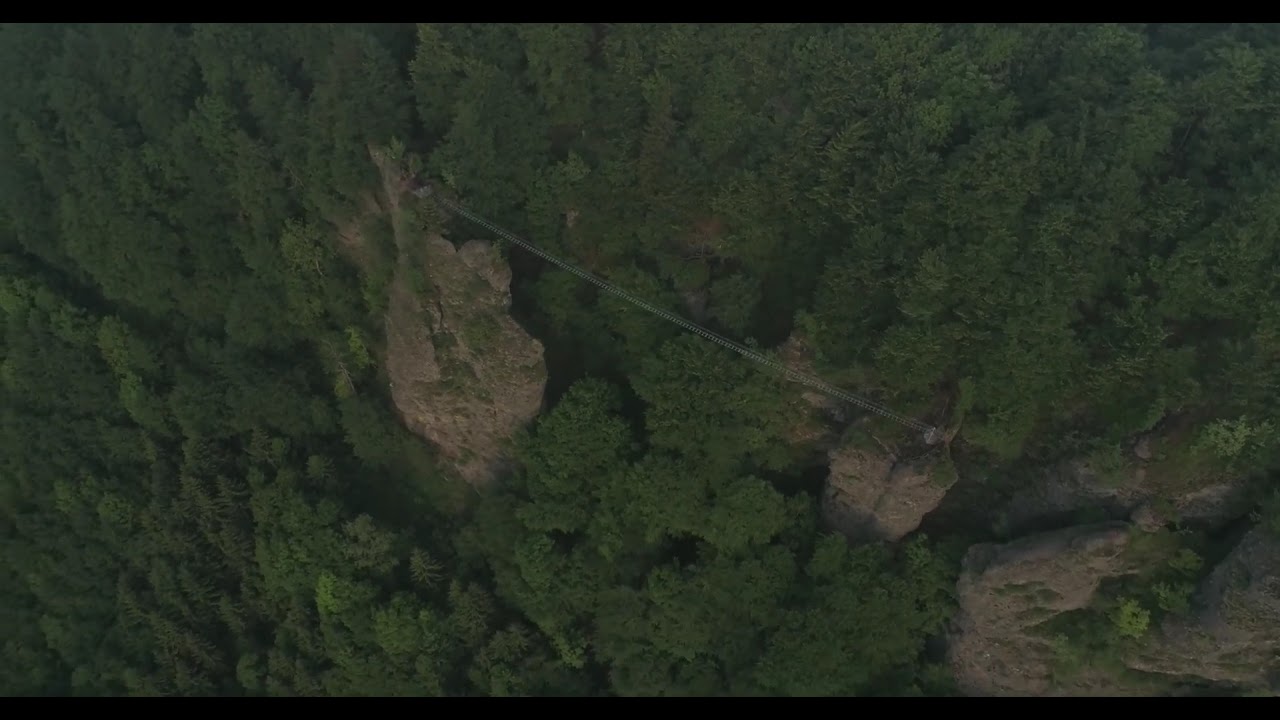In this aerial image taken during the daytime, we see a dense forest comprised of both deciduous and coniferous trees. At the center, tall, jagged rock formations protrude from the ground like fingers, cutting through the sea of treetops. These rocky outcroppings are connected by a series of wires, which appear to be a narrow, single-person bridge, likely a rope bridge. The scene, captured with a thin black header and footer but no side borders, appears dark with minimal bright light, adding a sense of mystery to the jagged cliffs and surrounding forest.